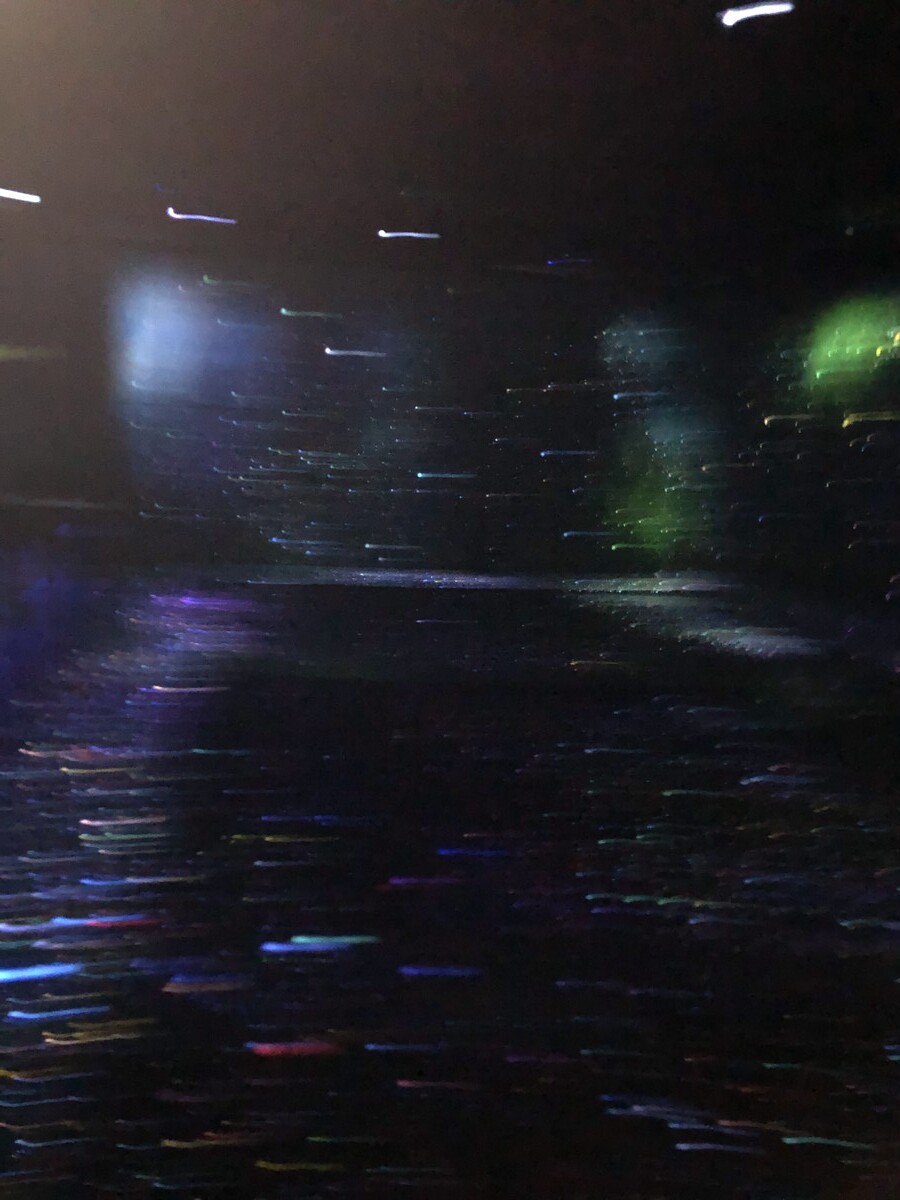This nighttime image features a kaleidoscope of colors, enveloping a room in a blur of light. The scene suggests the presence of a revolving disco ball, casting vivid reflections on the floor and walls. Dominating the top of the image are three larger white streaks, while the bottom is defined by more strikingly vibrant hues. A concentrated patch of green catches the eye on the right side, juxtaposed by a similar concentration of blue on the left. The lower half brims with streaks of green, red, purple, pink, and yellow, creating a mesmerizing and energetic display. The streaks become finer and less distinct toward the top, adding a sense of depth and dynamism to the image.